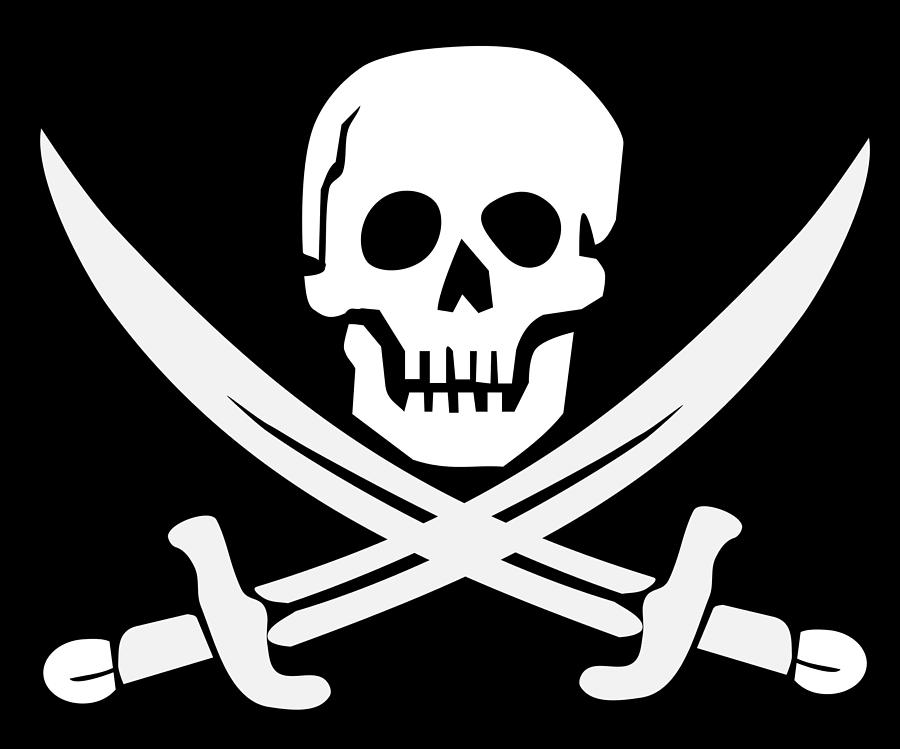The image is a black-and-white computer graphic clipart depicting a stylized pirate symbol. At the center top of the illustration is a smooth-textured skull with distinct dark eye sockets, giving it a haunting appearance. The skull features five top teeth and four evenly spaced bottom teeth, with a closed jaw that gives it a slight smile. Notably, there are cracks on the left side of the skull near the ear and a slight groove on the right side, as well as an uneven nose hole, with the right part larger than the left.

Beneath the skull are two crossed swords, substituting for the traditional crossbones often seen in pirate flags like the Jolly Roger. These swords resemble sailor cutlasses with curved blades and detailed hilts, pointing diagonally towards the upper corners of the rectangular image. The point where the swords intersect forms a prominent white diamond shape. The entire illustration is rendered in white against a stark black background, creating a striking and classic pirate-themed design.